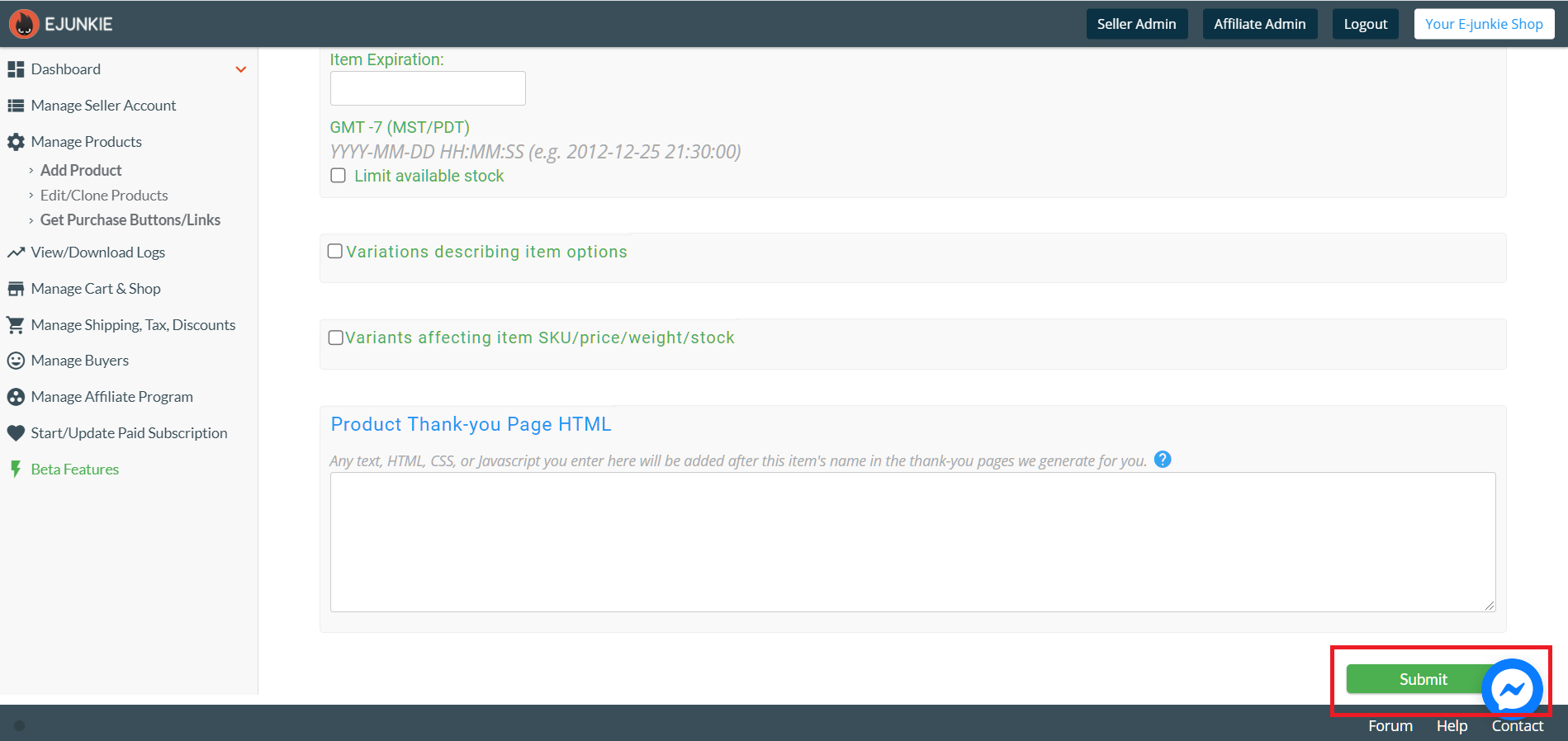The image displays a screenshot of an application interface, starting with the header and moving into the body and sidebar sections. 

**Header:**
- **Upper Left Corner:** Features the branding "e-junkie" alongside a striking logo with a red background and a fiery black design.
- **Upper Right Corner:** Contains several functional buttons:
  - "Seller Admin" (black background, white text)
  - "Affiliate Admin" (similar style)
  - "Logout" (button)
  - "Your e-junkie Shop" (white background, light blue text)

**Sidebar (Left Section):**
- A vertical list of navigational links, each accompanied by an icon and dark blue or dark gray text:
  - "Dashboard"
  - "Manage Seller Account"
  - "Manage Products"
  - "Download Logs"
  - "Manage Cart and Shop"
  - "Manage Buyers" (distinctly marked with a black smiley face icon)

**Main Body (Right Section):**
- Contains interactive elements such as:
  - Checkboxes next to labels with green text
  - "Variations": Describing item options (checkbox is empty)
  - "Variations Affecting Item SKU, Price, Weight, Stock"
- Below these options, there's a section titled "Product Thank You Page HTML" in blue text, followed by a multiline input field for typing text.
- In the bottom right corner, a conspicuous green "Submit" button with white text and a red outline is present. Additionally, there is a Facebook Messenger button situated beside the submit button.

This comprehensive layout combines various navigational and interactive elements, offering a detailed look into the application's usability and organizational structure.